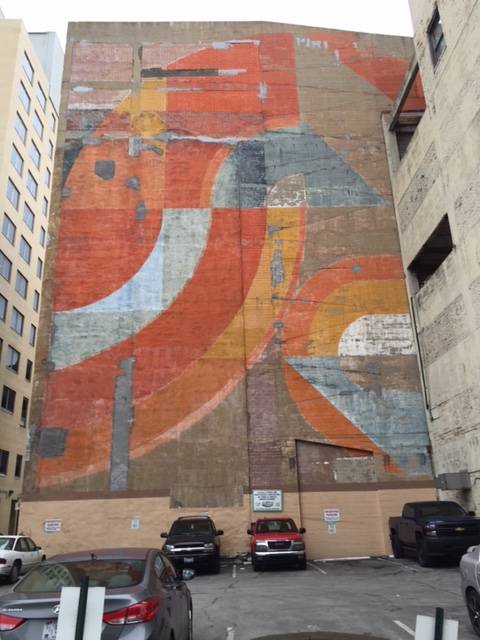The vertically oriented image captures an outdoor scene in an older-looking parking lot adjacent to the side of a tall building. The charcoal-gray parking lot is marked with white lines for parking spaces, though the paint is worn in places. In the lower left corner, a gray sedan is partially visible, showcasing its back end. Moving upwards and centered, three trucks are backed into parking spaces against the wall.

The wall itself features a large, abstract mural that extends from a lighter brown base to the top of the building. The mural includes organic, curved shapes in hues of orange, mustard yellow, blue, red, and white, some resembling a leaf, a track shape, and a pie wedge. The paint on both the mural and the wall shows signs of aging, with chipped and worn areas. The top part of the building displays additional worn brown stone.

To the left of this building, there’s a newer, light tan structure, approximately ten stories high, with numerous small square windows.

In the parking lot, a variety of cars are seen: in addition to the aforementioned gray sedan, there’s a blue pickup truck, a red car, a black car, a white car, and another vehicle that appears to be silver. Additionally, a faintly visible car with just its bumper or boot showing is located in the lower right corner of the image.